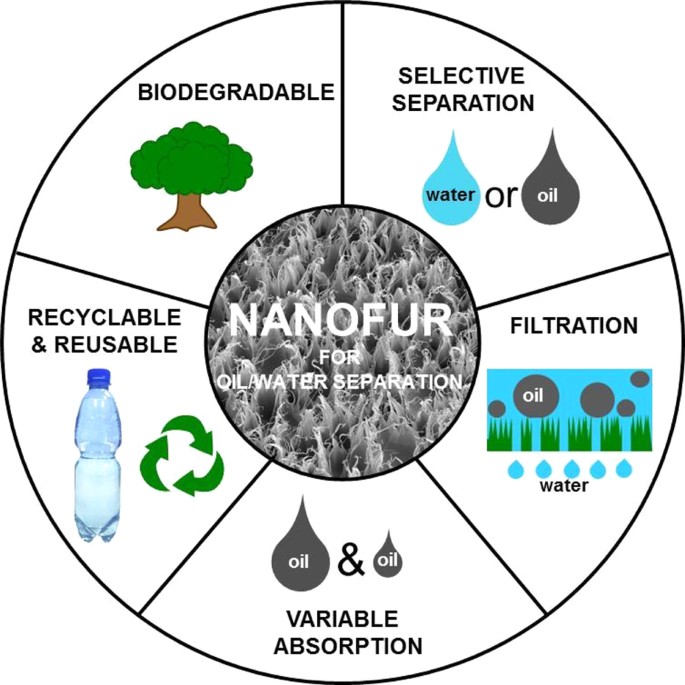The image displays a detailed, hand-drawn circular chart divided into five sections, all outlined in black. At the center of the chart, surrounded by an inner black circle, is a depiction of gray, web-like structures labeled "Nanofur for oil-water separation" in white font. 

Starting from the upper right at 1 o'clock, the first section, labeled "Selective Separation," features illustrations of two drops—one blue for water labeled "water" and another black for oil labeled "oil." The next section, positioned at 4 o'clock, is labeled "Filtration" and also depicts oil and water drops as an example. At the bottom section, aligned at 6 o'clock, it is labeled "Variable Absorption," showcasing a large oil drop and a smaller oil drop with an ampersand between them. At 8 o'clock, the section "Recyclable & Reusable" is illustrated with an image of a plastic bottle and a recycle symbol. Finally, at the upper left at 11 o'clock, the section "Biodegradable" is represented by the image of a tree.

The chart is visually clear and well-illuminated, providing an informative and concise breakdown of the various features and functionalities related to nanofur technology for separating oil and water.